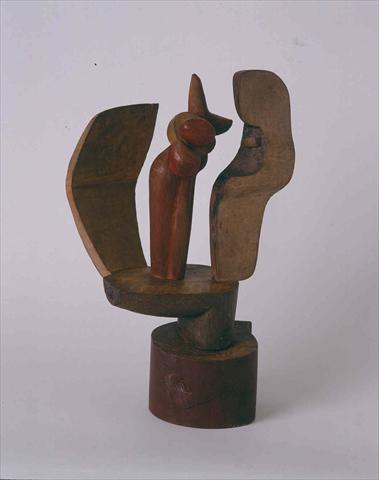This detailed photograph captures an abstract wooden sculpture set against a white background. The unique piece stands on a dark brown, cylindrical base and extends upwards to a wider, intricate form. Emerging from the base is a dark brown platform, upon which rests a striking silhouette that resembles a person or possibly an animal clad in a long red dress with a pointed hat, seemingly leaning forward. Flanking this central figure are two distinct wooden structures. To the left, there's a curved board, and to the right, a shape that intriguingly mimics a human ear. The sculpture, rendered in monochromatic wood tones of tans, reds, and deep browns, is subtly lit, emphasizing its complex textures and forms. The backdrop, a clean white, allows the intricate details and craftsmanship of the wooden sculpture to stand out vividly.